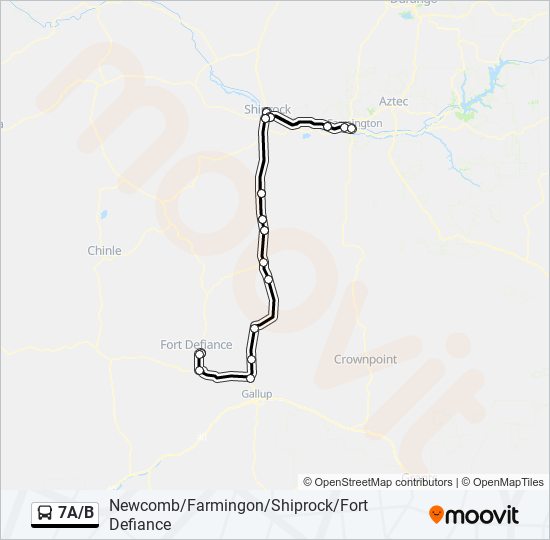This image is an aerial, bird’s-eye view transit map designed in a drawing style with a blue background, overlaid with a watermark reading "M-O-O-V-I-T" which spans diagonally from the top left to bottom right. The map outlines a bus route labeled 7A/B, marked by a bus icon. It illustrates a journey beginning at Fort Defiance, traveling southward and then eastward in a J-shaped path. Notably, the route passes through several key cities including Newcomb, Gallup, Crownpoint, and Shiprock, eventually reaching Farmington. Additional cities such as Lexington and Aztec appear along the path. Black outlines and dots help in tracking the route, while captions including city names and tiny area indicators are featured for clarity. The map, produced by Moovit, credits OpenStreetMap Contributors and OpenMapTiles, and it is adorned with an orange teardrop graphic in the bottom right corner. The depicted water body and various colored roads offer a spatial context to the viewer.